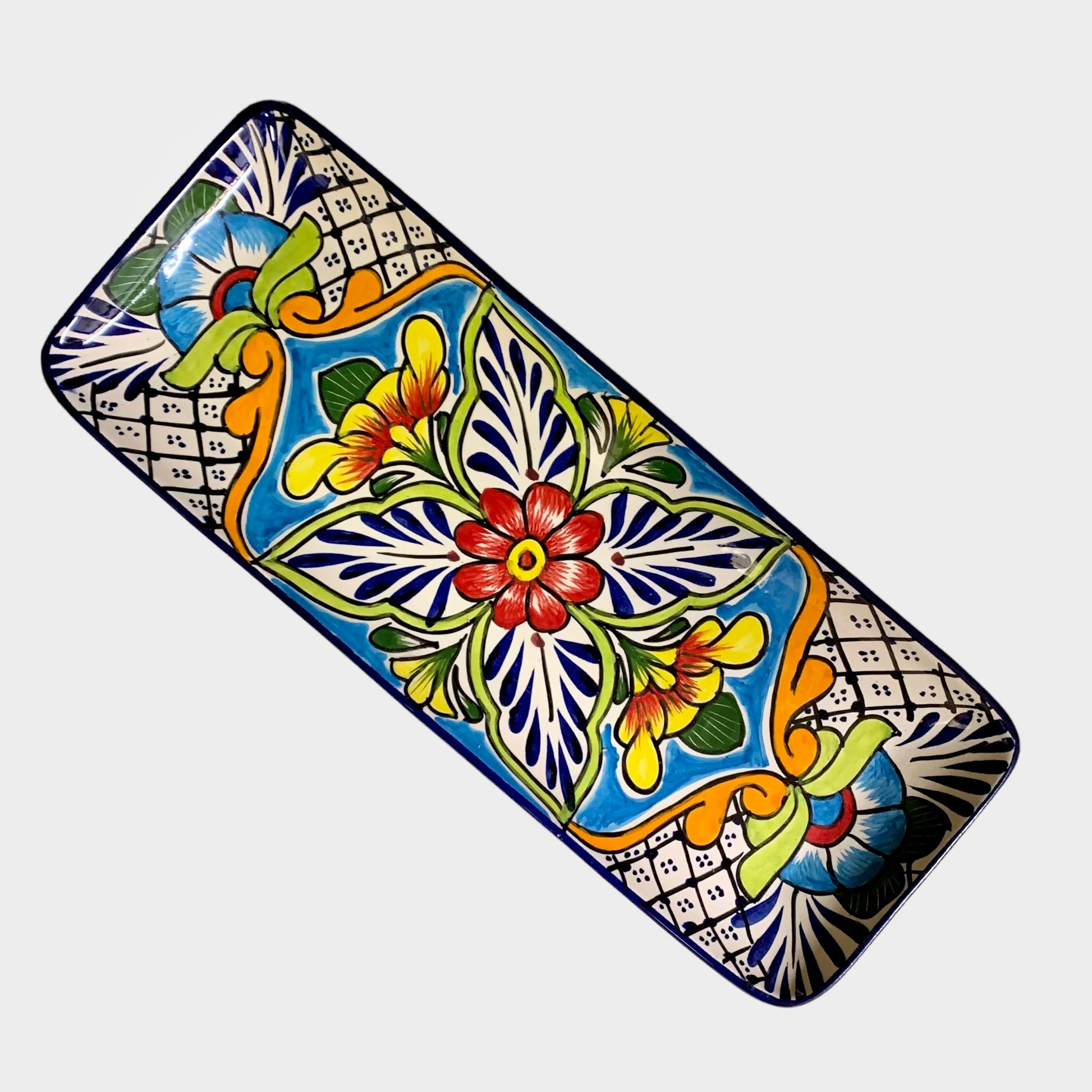This photograph showcases a rectangular, hand-painted serving tray, artfully arranged on a solid white background. The tray is vibrant and lively, featuring a complex, multicolored design. Its surface is characterized by a diagonal net pattern composed of white lines intersecting with squares, each punctuated by blue dots. Central to the tray's decoration is a prominent floral motif. This flower has a radiant yellow center with red petals, encircled by navy blue leaves outlined in light green. The flower design is set against smaller floral elements that mirror each other along the tray's axis, creating a symmetrical aesthetic. Each corner of the tray features additional blue flowers with red centers, further enhancing its colorful and harmonious appearance. The entire scene is a testament to intricate craftsmanship, making the tray a striking centerpiece suitable for decorative or functional use.